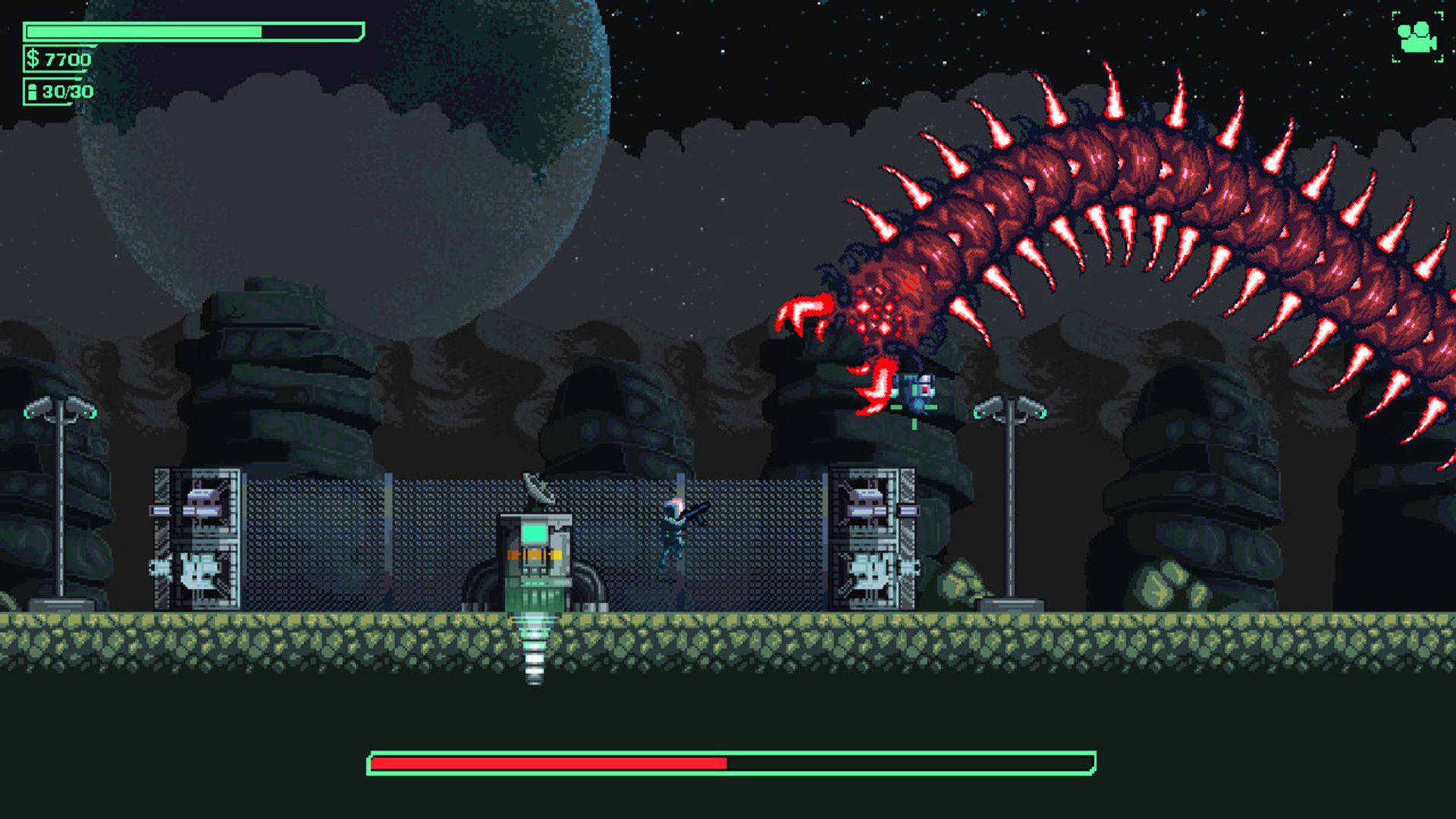The screenshot is from an old-school side-scroller video game with a retro aesthetic that seems to be a nod to classic Super Nintendo titles, possibly resembling but not quite identical to games like Contra. This sci-fi shooter features a current battle scene against a massive red centipede-like boss, which has antler-like projections and numerous segmented body parts, accented in shades of red and wine. The centipede is positioned on the right of the screen, hovering above the ground and facing the playable character in the middle, a female protagonist with striking pink hair, armed with a gun. The game's user interface shows the boss's health bar at the bottom, which is currently at half capacity, and the player's health in the top left corner, indicating three-fourths health remaining. The setting is outdoors, with a large plant visible in the background, a gray moon in a starry black sky, and additional environmental details such as a light pole, trees, and a satellite dish pointing skywards, all contributing to the game's sci-fi atmosphere.